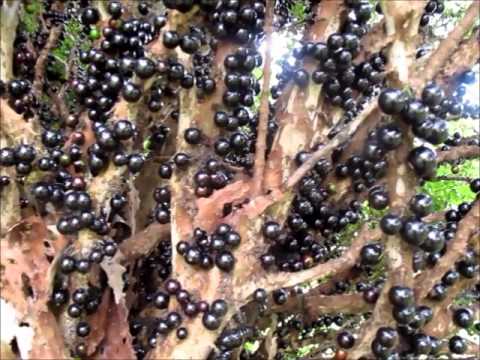This image depicts a detailed close-up of a tree adorned with an array of shiny, round berries. The berries, primarily a deep purple-black, exhibit some variations in color, including hues of dark burgundy, purplish tones, and a few with a silver cast. The plant material features ridges of tan, pink, and white stretching out in multiple directions, with light streaming through, highlighting their shapes and textures against a bright sky backdrop. The irregular surface underneath the berries displays a spectrum of colors, ranging from bright fluorescent green to dark blues, whites, and grays, resembling tree limbs. In the background, hints of green foliage and grass are visible, adding to the natural vibrancy of this sunlit scene captured in the middle of the day.